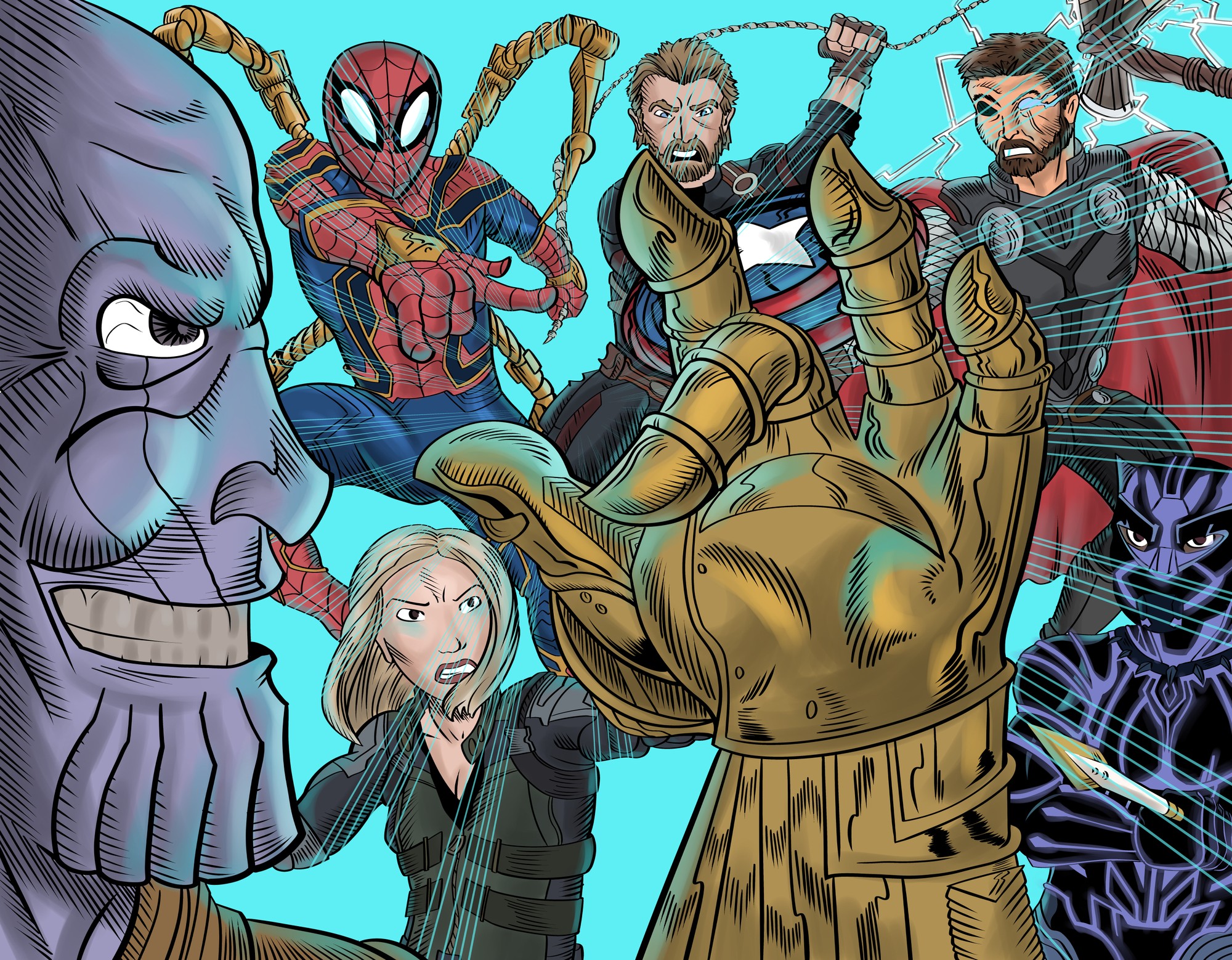This detailed and colorful cartoon illustration, likely a piece of fan art, captures an intense face-off between Thanos and several iconic superheroes, suggesting a scene inspired by Marvel's Avengers and Spider-Man. Thanos, prominently featured in the foreground, has a large, light and dark purple face with a menacing grin and is holding up his gauntlet with one finger down. Surrounding him are various superheroes: Spider-Man appears in his special suit with two mechanical arms extending from his back; Thor, equipped with an axe and missing one eye, stands next to Hawkeye, who holds a chain; Black Widow, with short blonde hair, looks fiercely determined between Thanos's head and glove; and Black Panther, shrouded in black with blue shadowing, is positioned in the lower right corner in his masked suit. Additional characters, such as one dressed in blue and red, one in all black, and another in black with a red cape, further populate this vividly detailed scene. This striking illustration was most likely created using a digital graphic imaging program, showcasing the artist's skillful blend of drawing and painting techniques.